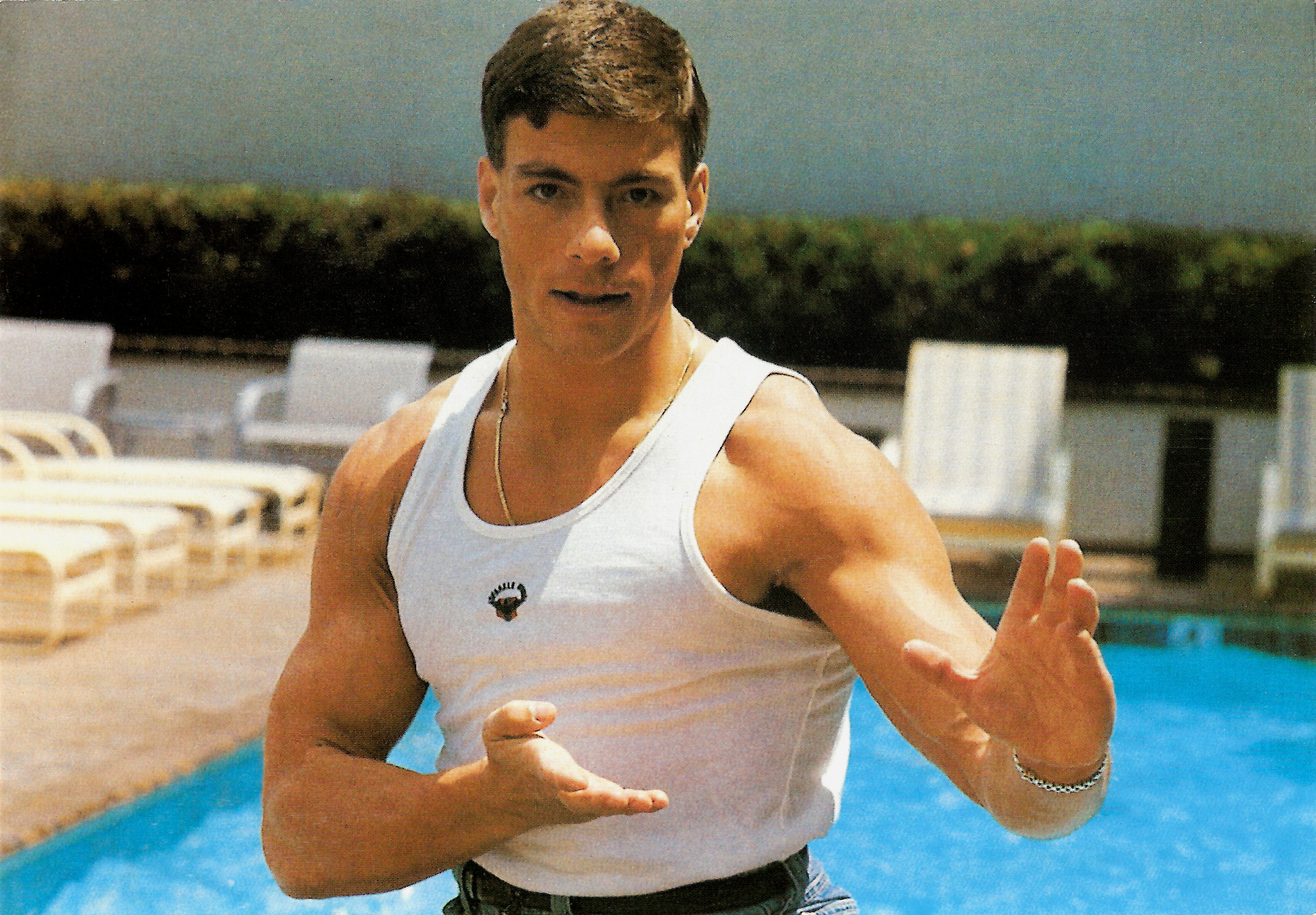This is a detailed color photograph of a muscular man striking a karate pose by a swimming pool. The man, who resembles Jean-Claude Van Damme, stands waist-up in the center of the image. He has short brown hair parted to the side and is looking directly at the camera. He is wearing a white tank top with a small black logo on the front, a gold necklace, and a silver bracelet on his left wrist. His right arm is bent at the elbow with his fist near his chest, while his left arm is extended towards the camera with his palm raised. The background features a blue swimming pool to the lower right and white lounge chairs to the left and behind him. Additionally, there is a green hedge and a white wall above the hedge, framing the poolside setting. The colors in the image include blue, white, tan, red, green, and black.